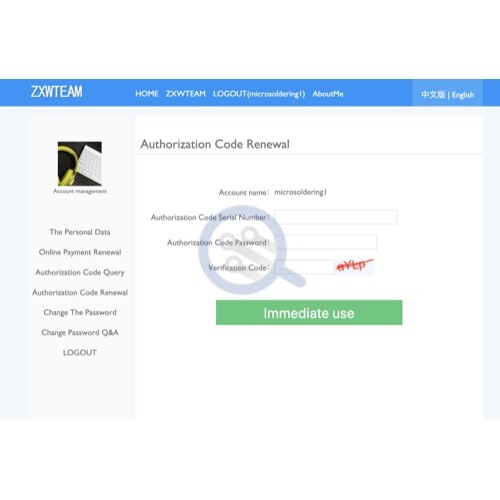A web page for the ZXW team displays a structured and user-friendly interface. At the top, the website features the title "ZXW Team" with navigation tabs including "Home," "ZXW Team," "About Me," and "Logout." There's also an option to change the language in the top right-hand corner. The left sidebar presents a vertical menu with links for "Personal Data," "Online Payment," "Review Authorization Code," "Authorization Code Renewal," "Change Password," "Q&A," and "Logout."

The central focus of the screen is the "Authorization Code Renewal" section. Here, users are prompted to fill in several fields: "Account Name" with a corresponding input box, "Authorization Code Serial Number" with another input box, "Authorization Code Password," and "Verification Code," each with its respective input box. At the bottom of this section, there is an "Immediate Use" button to confirm the renewal process.